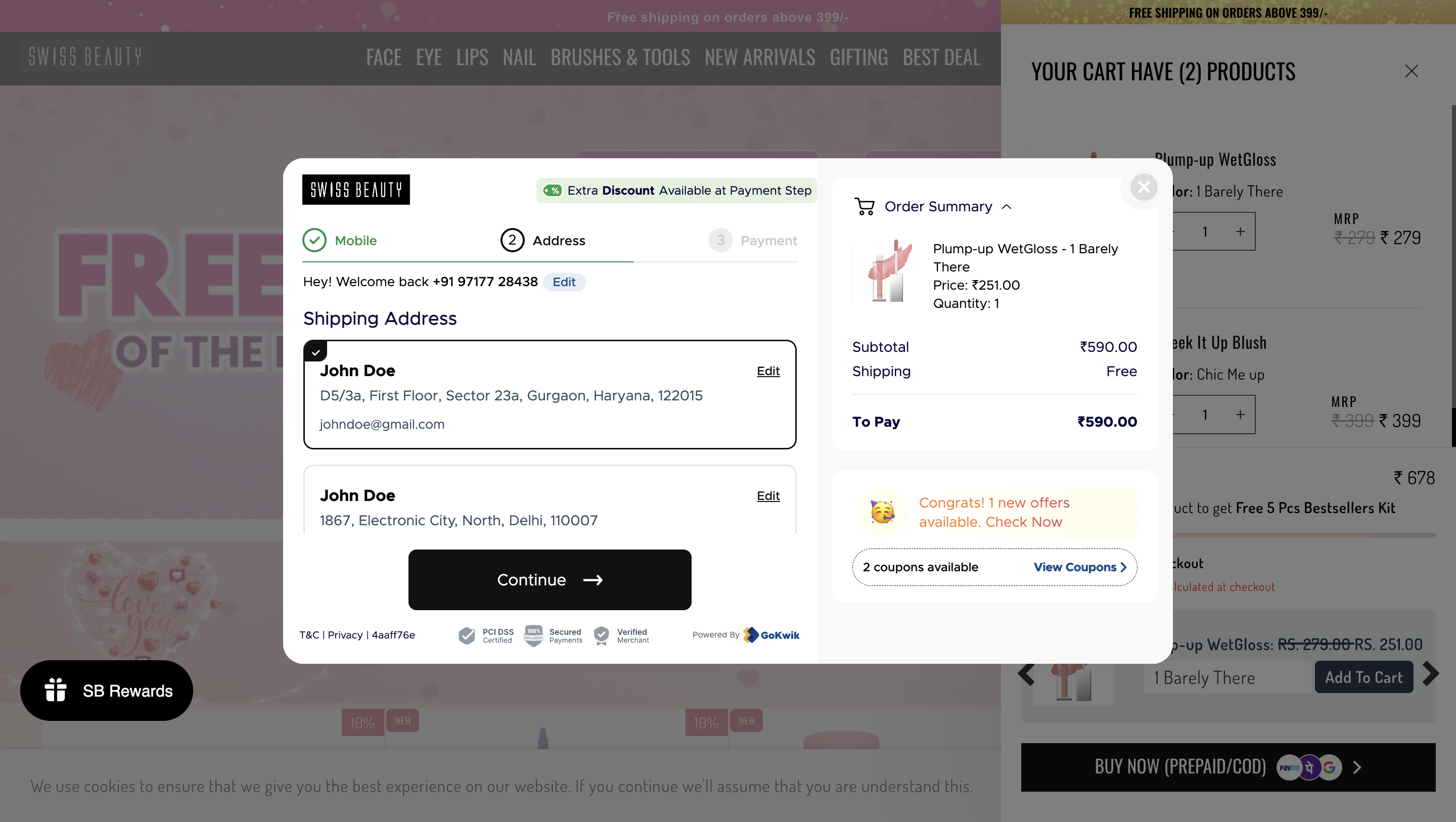The image showcases a detailed interface of an online shopping platform for Swiss Beauty products. The background prominently features the brand name "Swiss Beauty" along with navigation categories: Face, Eyes, Lips, Nail, Brushes and Tools, New Arrivals, Gifting, Best Deal, and Free Shipping on orders above $399. 

In the foreground, a screen indicates that the user's cart contains two products: one item priced at $279 and another at $399, leading to a subtotal of $678. Below this, options to "Buy Now" or use a "Pre-Pay Code" are available.

An overlaying screen offers an additional discount during the payment step and prompts for mobile, address, and payment details. The message "Hey, Welcome Back" is followed by a partially obscured phone number, 919-177-28433, and an "Add" button for adding information. The shipping address displayed is John Doe, DS-3S, First Floor, Sector 23A, Guaran-Hariyana, 122015, alongside the user's email details. A black "Continue" button is visible at the bottom of the screen.